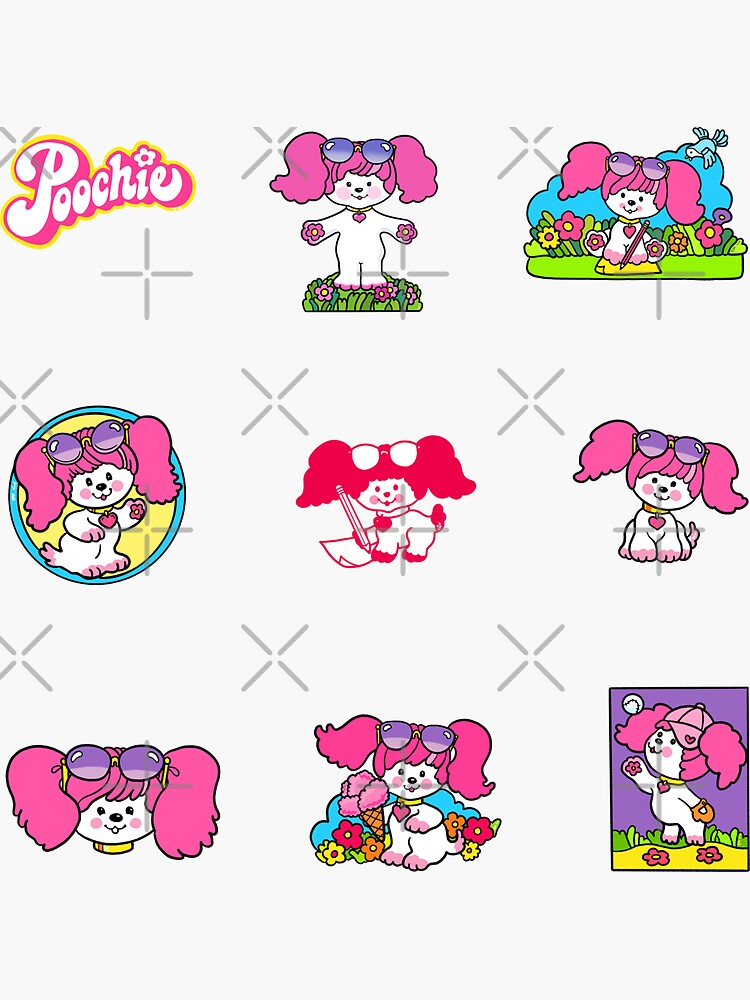The image showcases a series of nine distinct cartoon-like illustrations of a character named Poochie, presented on a light gray background adorned with line-drawn X's. At the top left corner, the character's name, "Poochie," is highlighted in a comic book-style, bubbly white text with a hot pink background. This playful character resembles a white dog with fluffy, curly pink hair, including hot pink bangs and long ears. Poochie is often seen with purple sunglasses on top of its head, though in one illustration, it sports a pink baseball cap with a red heart.

The illustrations depict Poochie in various activities and poses, showcasing its cheerful personality. The first image features Poochie standing upright with arms outstretched in a hug-like motion, standing amidst flowers. The character continues to exhibit different poses in subsequent images, including smiling in front of flowers, outlined with a blue ring, appearing with red accents while drawing, and sitting down with glasses on its forehead. In another illustration, only Poochie's face is visible, demonstrating a close-up view. Additional scenes show Poochie playing with objects surrounded by flowers and standing on its hind legs with a raised paw, set against a purple background. This detailed depiction of Poochie highlights its whimsical nature and vibrant pink and white color scheme.